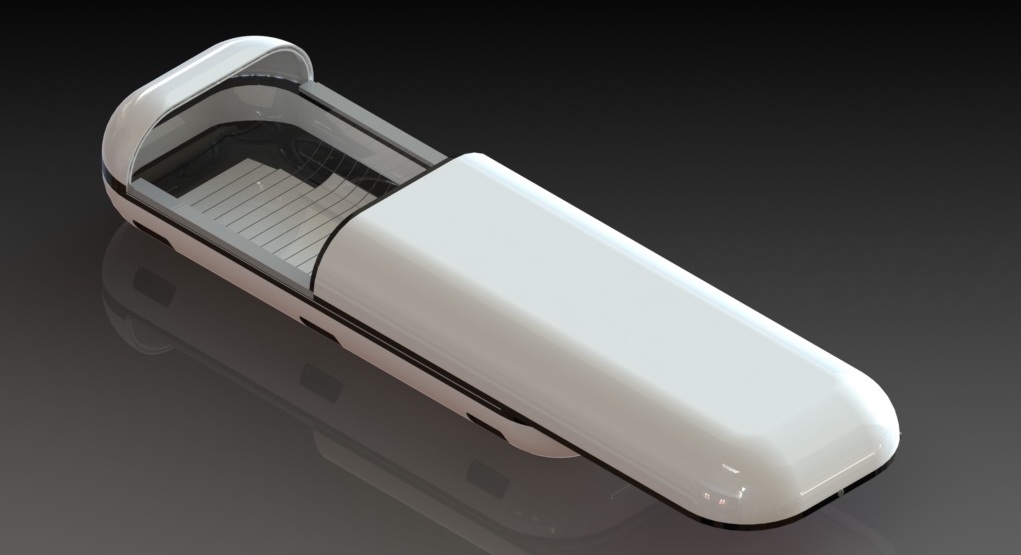The image showcases a digitally-rendered, futuristic device that bears a resemblance to a sensory deprivation tank or a modernized casket. The setting appears to lack any scale references, making it ambiguous whether the device is as large as a person or as small as a tic-tac container. The device itself is predominantly white with black borders and black windows on its sides. It is positioned on a reflective, gray surface, which mirrors both its shape and features. The top of the device slides open, revealing a hollow interior lined with a black surface. Inside, there is a white mat with gray pinstripes, resembling loose-leaf notebook paper. The background of the image is a dark green color, adding to the futuristic and somewhat mysterious ambiance of the scene.